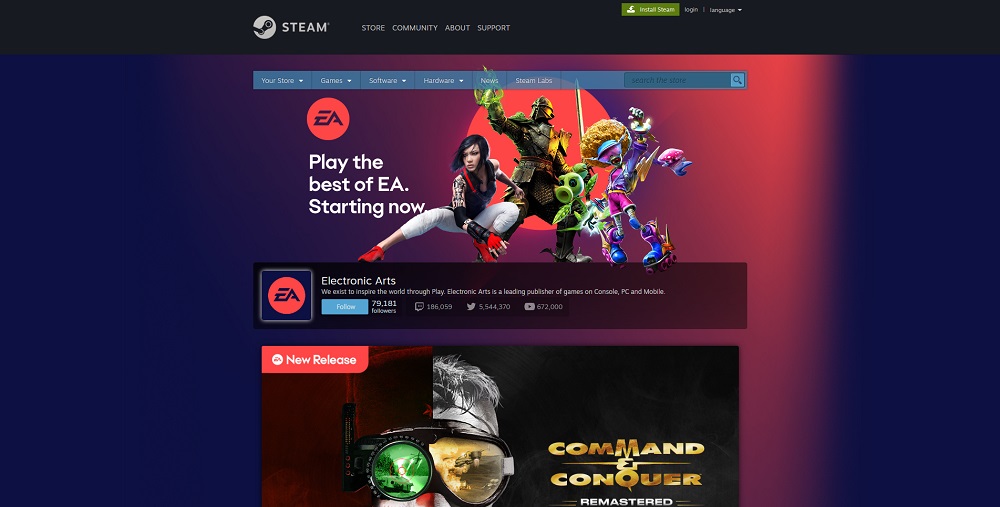The image displays a detailed interface of the Steam platform, featuring tabs such as "Store," "Community," and "Support" at the top. The interface is presumably shown in a South Asian language. Highlighted categories include "Games," "Software," "Hardware," and "iOS Team Labs." 

A search bar with a magnifying glass icon is visible for easy navigation. An orange circle indicates that EA (Electronic Arts) games are currently featured, prompting users to "Play The Best of EA Now." Additionally, a red circular element is in the background.

In the foreground, a woman crouches, likely a character from the game "Mirror's Edge." Other elements in the scene include a person with an afro, a plant, and a colorful pink or purple background. 

A rectangle highlighting "Electronic Arts" describes the company's mission to "inspire the world through play," noting its position as a leading publisher for console, PC, and mobile games.

There are numbers displayed, possibly indicating statistics or identification codes: "1860495044070," "672000," and a price tag "$99000" alongside a note about a new mobile phone.

Lastly, a red rectangle signifies "New Releases," and on the left, goggles appear to suggest VR or AR capabilities, featuring titles like "Command and Conquer."

Overall, the image integrates various elements of the Steam platform with specific emphasis on EA's offerings and featured characters from popular games.